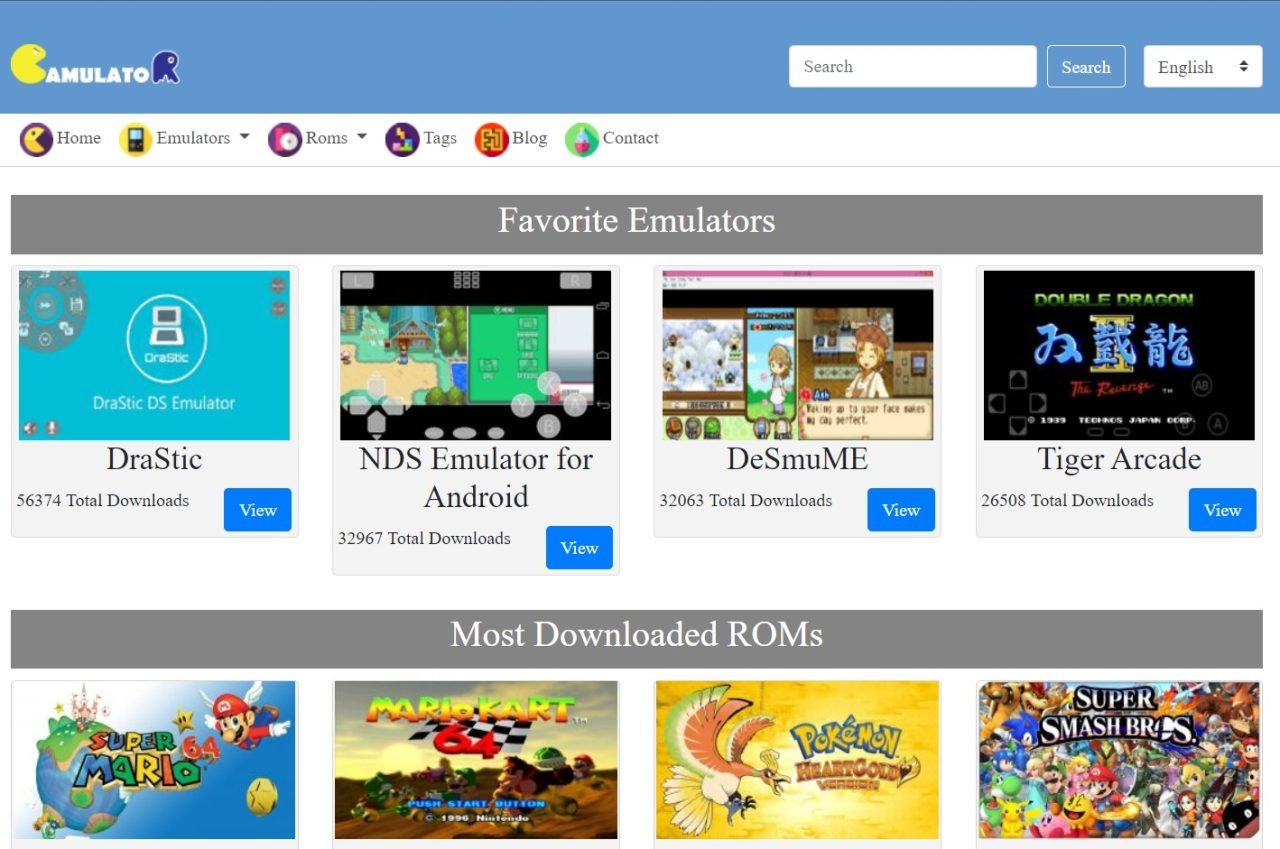The image showcases a vibrant and colorful website from "MyEmulator," featuring a playful yellow Pac-Man shape on the left and a purple gorilla on the right. At the top of the page, there is a white search bar where users can easily input search queries and hit the search button. The site is presented in English and includes a drop-down menu with tabs labeled: Home, Emulators, ROMs, Tags, Blog, and Contact, each accompanied by an icon.

On the left side of the screen, within a gray bar labeled "Favorite Emulators," there are four clickable boxes featuring different emulator options. The first box is titled "drastic" and includes information about its total downloads, with a blue "View" button to access more details. The second box displays the "NDS emulator for Android," also offering a blue "View" button for more information. The third box, labeled “DeSmuME,” features an image of a cartoon character and provides viewing options. The fourth box is titled "Tiger Arcade" and is highlighted with Asian writing.

Adjacent to these boxes, two images capture attention: one showing a stylized blue computer icon within a circle, and the other displaying a general computer image of a video game. Below the emulator section, the site lists "Most Downloaded ROMs," showcasing popular games such as Mario Brothers, Mario Kart, Pokemon, and Super Smash Brothers.